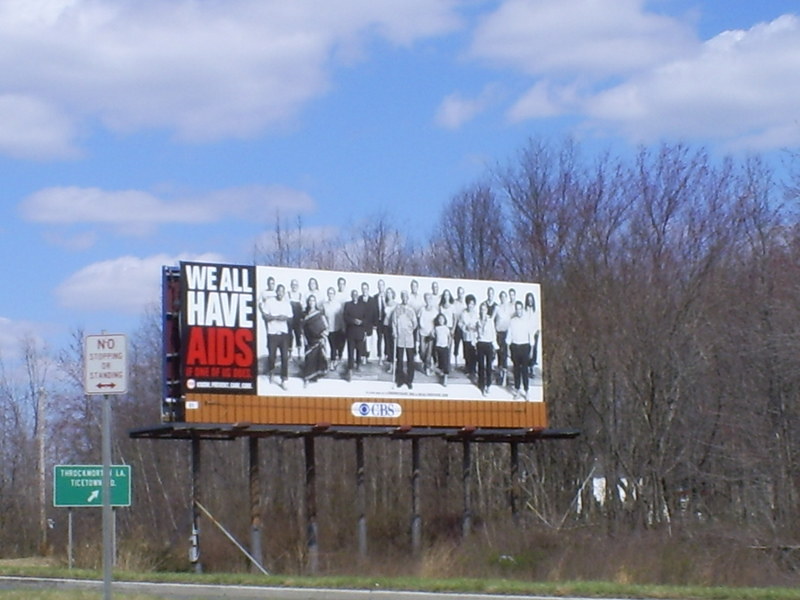The photograph captures a striking billboard positioned at the edge of a highway against a backdrop of a clear blue sky dotted with white fluffy clouds. Surrounding the billboard are dense, leafless trees with a mix of brown and gray trunks, indicative of a seasonal transition. Below the trees, green grass frames the roadside scene.

The billboard prominently features a black rectangle on its left side with the impactful message in white letters reading "We all have," followed by "AIDS" in bold red letters. The top portion of the billboard showcases black-and-white images of people from diverse races, ages, and backgrounds, standing together as a symbol of unity and awareness.

Adjacent to the base of the billboard, a brown section marked with vertical lighter brown lines houses the CBS logo. Additionally, there's a small, rectangular road sign on a silver pole to the left of the billboard, with red writing that is partially obscured. The overall scene captures a poignant and unifying message aimed at raising awareness about AIDS in a tranquil outdoor setting.